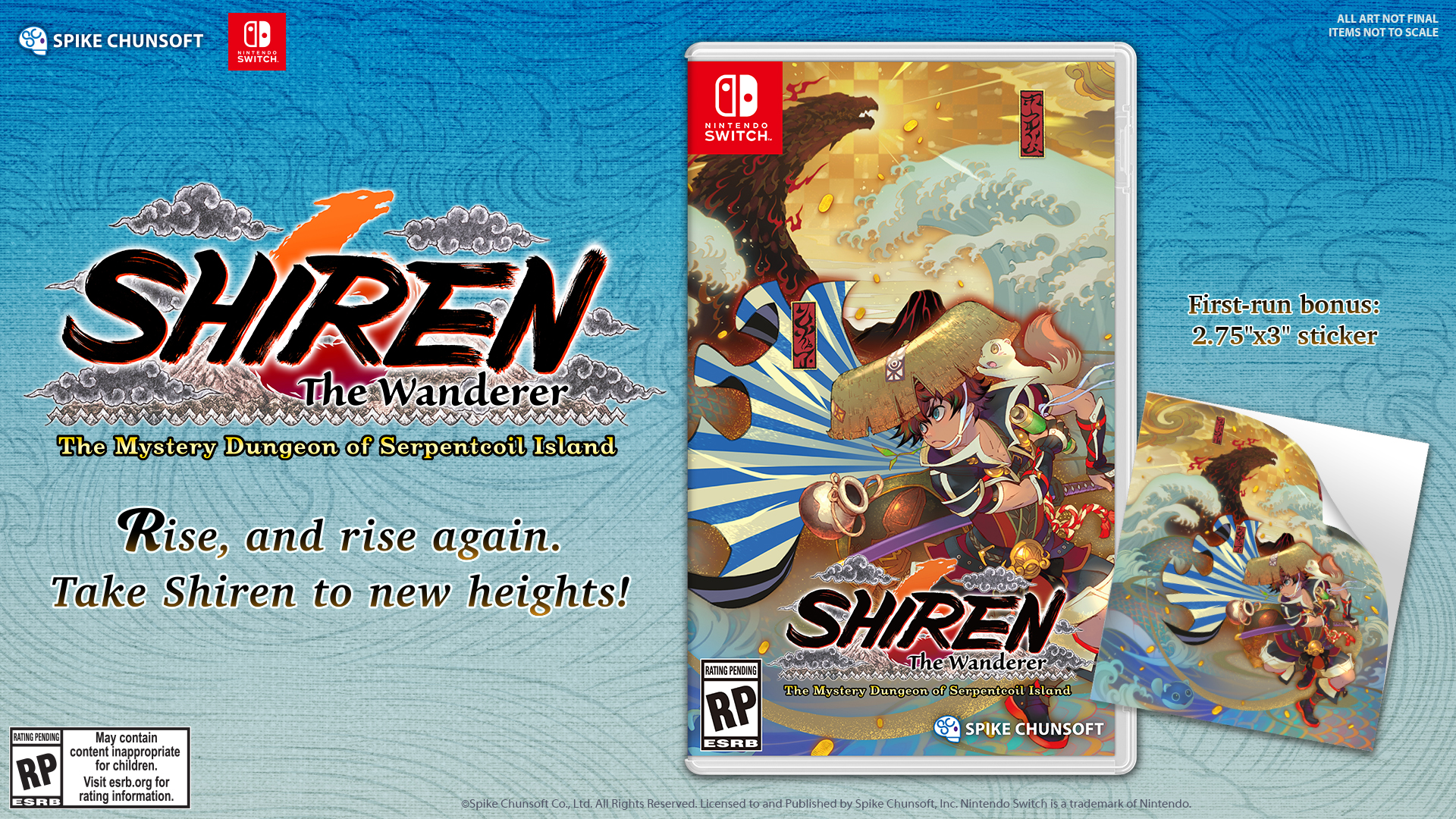This is a detailed advertisement for a Nintendo Switch video game titled "Shiren the Wanderer: The Mystery Dungeon of Serpent Coil Island." The centerpiece of the image is a Nintendo Switch game case featuring a vibrant cover. The cover depicts an intricate Japanese-style artwork with large ocean waves, a tree with Asian writing, and a male character dressed in black and red clothing with a white cat perched on his shoulder. The character appears to be in an adventurous scene reminiscent of classic Japanese art, potentially hinting at the game's thematic elements.

On the left side of the image, the game's logo is prominently displayed in a big black font, "Shiren the Wanderer," with a smaller yellow font underneath that reads "The Mystery Dungeon of Serpent Coil Island." Below the title, the tagline, "Rise and rise again, take Shiren to new heights" is featured in a black font, adding a motivational call to action.

In the top left corner, the logos for Spike Chunsoft, the game's developer, and Nintendo Switch are visible, with a note in the top right corner stating, "All art not final, items not to scale." The bottom left of the image includes the rating pending (RP) symbol and a cautionary note indicating that the game may contain content inappropriate for children, urging viewers to visit esrb.org for more information.

Additionally, to the right of the game case, there's a highlighted feature stating "First run bonus: 2.75 inch by 3 inch sticker," accompanied by a smaller image of the sticker, which mirrors the game's main artwork. Overall, this advertisement effectively combines visual and textual elements to present a compelling snapshot of the game and its bonus content.